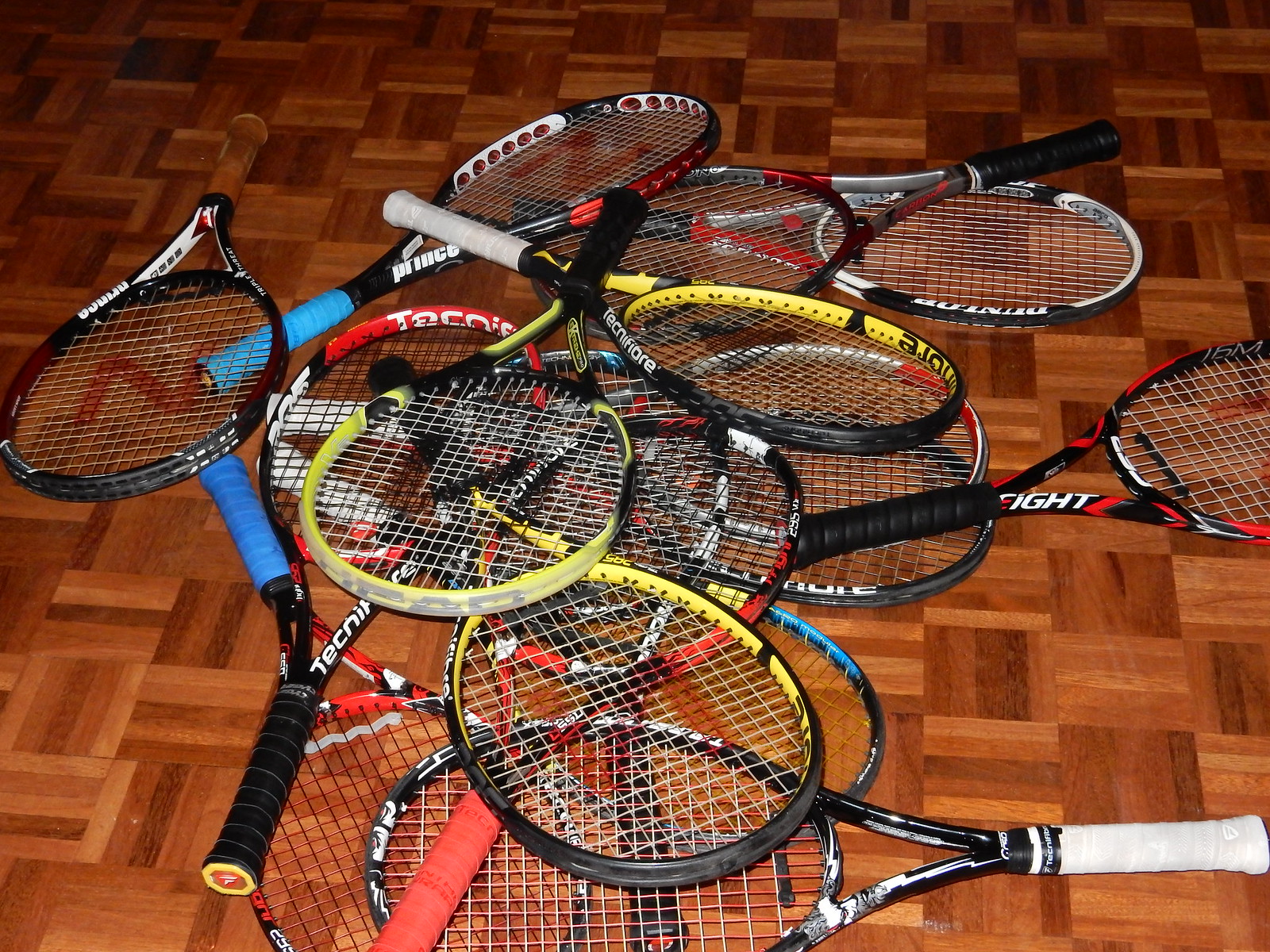This photo, likely taken indoors during the evening due to the dim lighting and the flash being the primary light source, showcases a haphazard pile of approximately 10 to 15 tennis rackets scattered on an intricate wooden tiled floor. The floor's tiles consist of square shapes made up of rectangular wooden strips arranged in different orientations, creating a pattern with varying shades of light brown. The tennis rackets, seemingly tossed onto the floor without any particular order, feature diverse brands and designs. While "Prince" is one identifiable brand, most others are hard to distinguish. The rackets have handles in assorted colors including white, black, blue, grey, and red. The metal parts of the rackets predominantly feature black in their design, with accents of yellow, red, or white. Notably, a red racket lies beneath a yellow one, with a blue one also in the same vicinity. The prominent racket in the right front corner has a white handle, adding to the colorful and chaotic ensemble on the wooden floor.